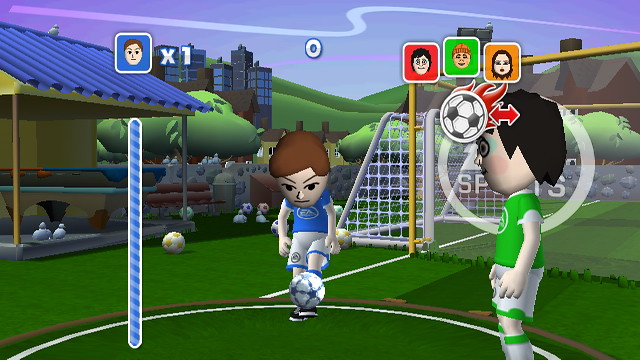The image depicts a scene from a video game designed in a 16-bit anime style, showcasing a soccer match. In the center left, a male player with brown hair, wearing a blue jersey and white shorts, is captured mid-action, focusing intently on the ball at his feet. On the right side, another player with dark brown or black hair is dressed in a green short-sleeved jersey and white shorts, complemented by white socks with green at the top, seemingly disengaged from his opponent. A white soccer goal and net are positioned behind this player to the right. Surrounding the players, the field features a distinct circle with a green center and white rim. In the backdrop, multi-story buildings and rolling green hills stretch under a purple sky marked by a white S-shaped line, hinting at some form of dynamic game element or weather effect. Additional game interface elements include three faces and a ball above the right player, likely indicating player selection options, a face with an 'X1' on the upper left side, and a score of zero at the top center. To the far left, a blue progress bar or line and some trees are partially visible, further contextualizing the scene within the game's environment.